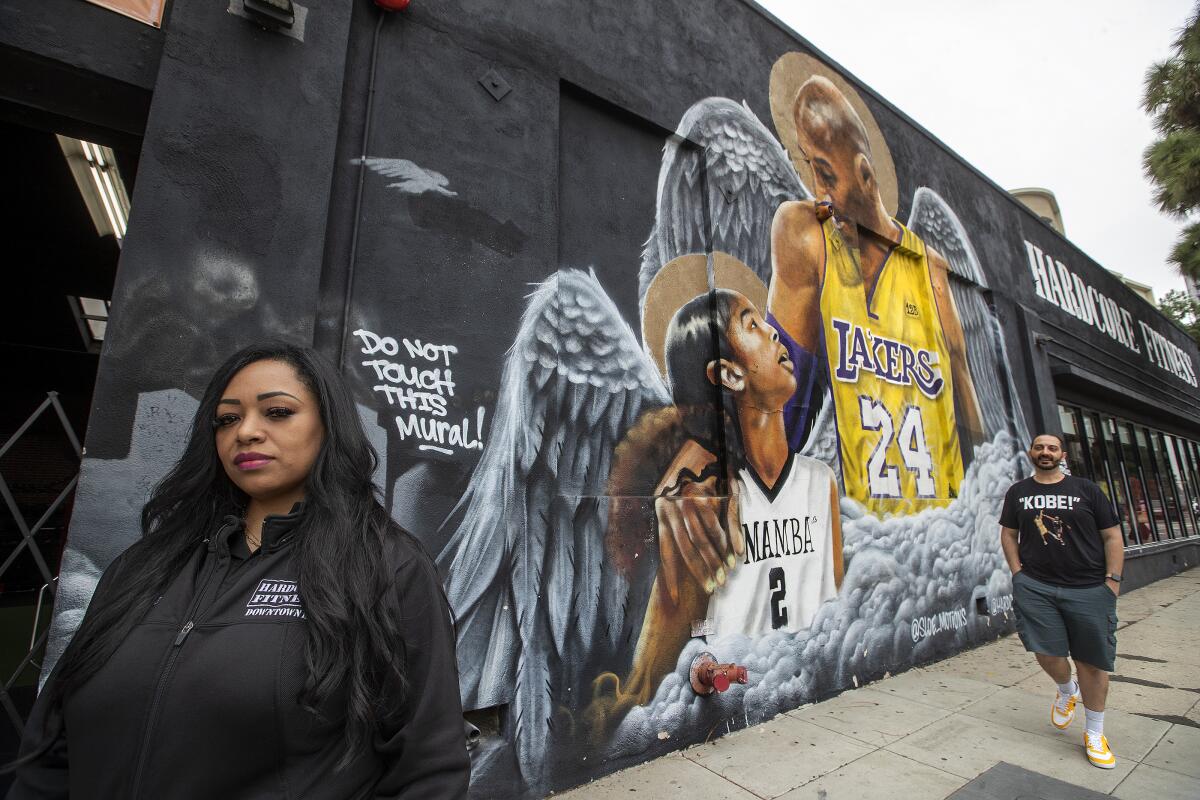This horizontally-oriented photograph captures an outdoor mural on a dark gray or black wall at the Hardcore Fitness Center. The mural is an evocative tribute to Kobe Bryant and his daughter Gianna, featuring lifelike paintings of the two adorned with angel wings and halos, likely created in their memory following the tragic helicopter crash. Kobe is depicted in his iconic Los Angeles Lakers basketball jersey, golden with blue lettering and the white number 24, as he tenderly rests his right arm on Gianna's shoulder. Gianna's gaze is directed upward toward her father, and she is dressed in a white "Mamba" jersey with a blue number 2.

Beside the mural, in white text, there is a clear instruction: "Do not touch this mural," underscoring its significance and encouraging respect. The scene is set on a clear day, with two people walking by on the adjacent sidewalk. On the lower left, a woman with long dark hair and dark skin, adorned with red lipstick, wears a Hardcore Fitness zippered jacket and looks directly at the camera. On the lower right, a man walks with his hands in his pockets, sporting a black short-sleeved t-shirt emblazoned with "Kobe!" in white letters, gray shorts, and white and yellow tennis shoes. The overall atmosphere reflects a moment of homage in a community-centered space.